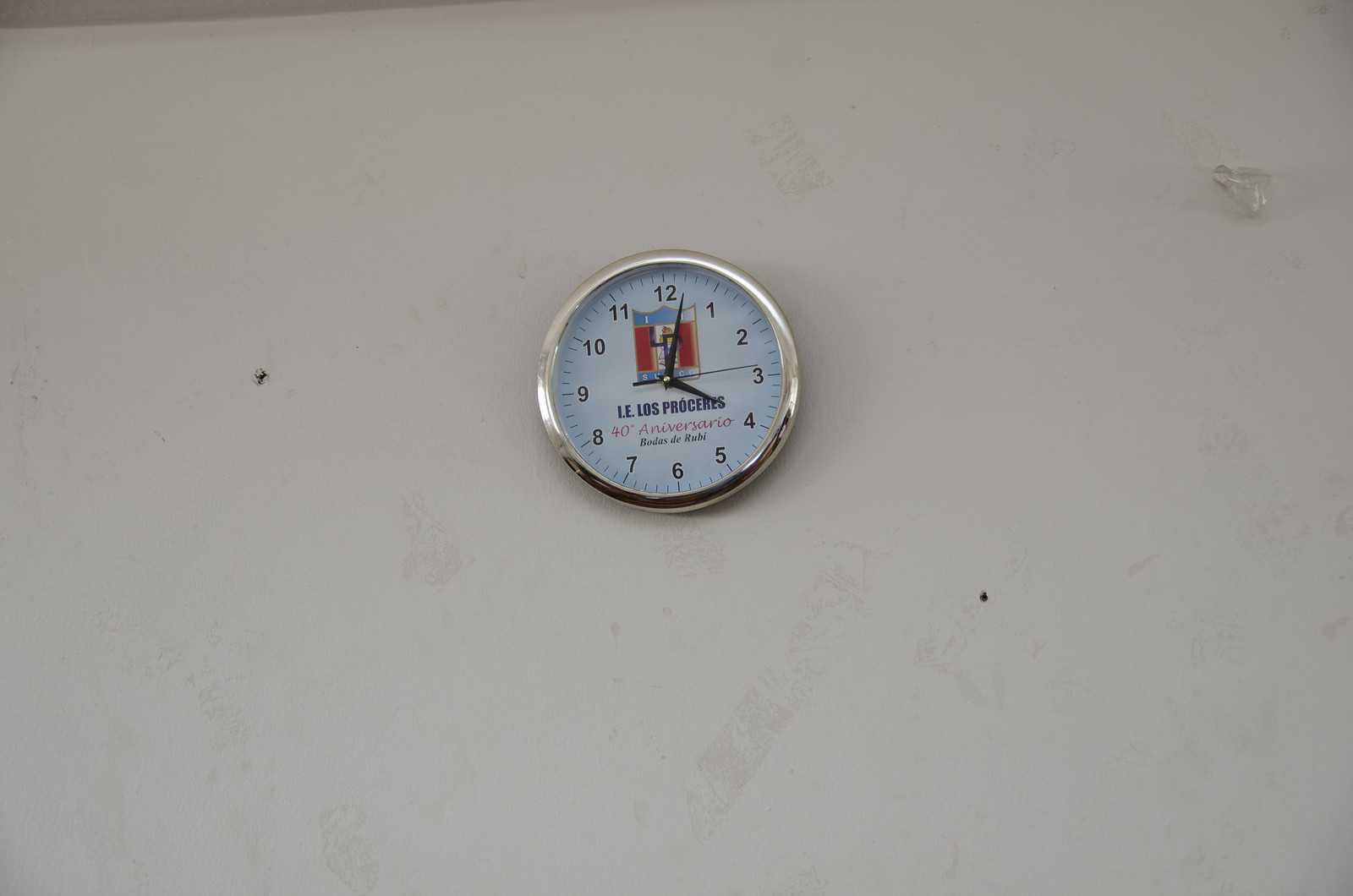This indoor photograph captures a slightly upward angle view of a wall clock mounted on a gray, somewhat blemished plaster wall, featuring several marks and holes, particularly to its left and lower right. The clock, encircled by a chrome bezel, showcases a white face with black numbers and minute markers evenly spaced around the dial from 1 to 12. The current time displayed is approximately 4:03, indicated by black hour, minute, and second hands – the latter positioned at the three o'clock mark.

Centered below the 12 o'clock position is a detailed crest or shield emblem. This emblem is divided into sections with a blue top, red vertical stripes on either side, and white central stripes, with the letters "L" and “P” possibly discernable within it. Adorned with gold outlines, the emblem exudes a regal quality.

Beneath the clock's center, in blue letters, is "I.E. LOS PROCERES," followed by a red script inscription reading "40th aniversario," and a lower section in blue that remains illegible. Additionally, the photograph hints at some clear mounting hardware in the upper right corner of the wall.